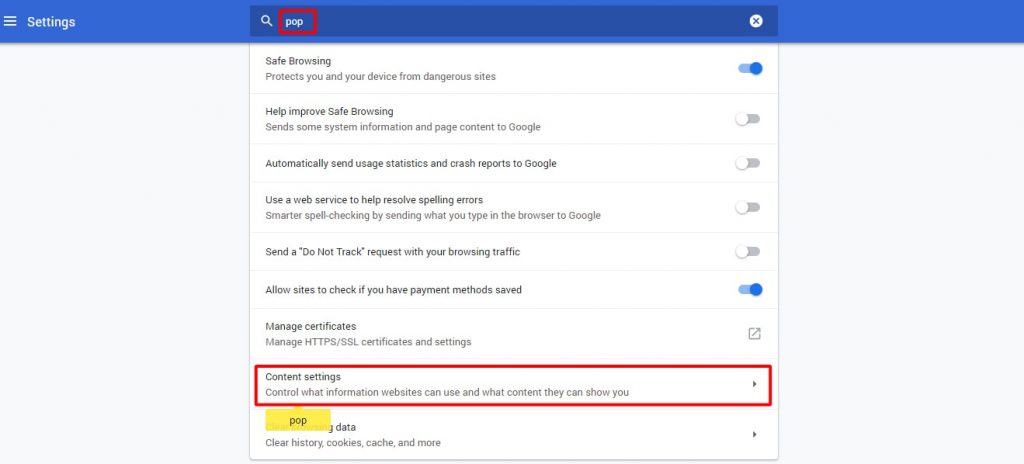**Detailed Caption:**

The image displays a settings page, identified by a narrow blue header bar at the top with the word "Settings." Near the top, there is a red-framed label that appears to read "PCP," though the letters aren't entirely clear. Below the header, the page itemizes various security and privacy settings.

The first entry, "Safe Browsing protects you and your device from dangerous sites," is toggled on, implying that this feature is active. The subsequent four settings are turned off:

1. "Help improve Safe Browsing: Send some system information and page content to Google."
2. "Automatically send usage statistics and crash reports to Google."
3. "Use a web service to help resolve spelling errors."
4. "Smarter spell checking: By sending what you type in the browser to Google."

Next, there is an option labeled "Send a 'Do Not Track' request with your browsing traffic," which is also turned off.

Following this, an active setting reads "Allow sites to check if you have payment methods saved," denoted by its toggled-on status.

The final setting listed is "Manage certificates: Manage your HTTPS/SSL certificates and settings," which is not turned on.

At the bottom of the page, within a red-outlined rectangle, there is a link to "Content settings: Control what information websites can use and what content they can show you."

Additionally, a small yellow rectangle contains the words "Top," "Data," and "Clear history, cookies, cache, and more," followed by a right-facing arrow indicating navigation to further options.